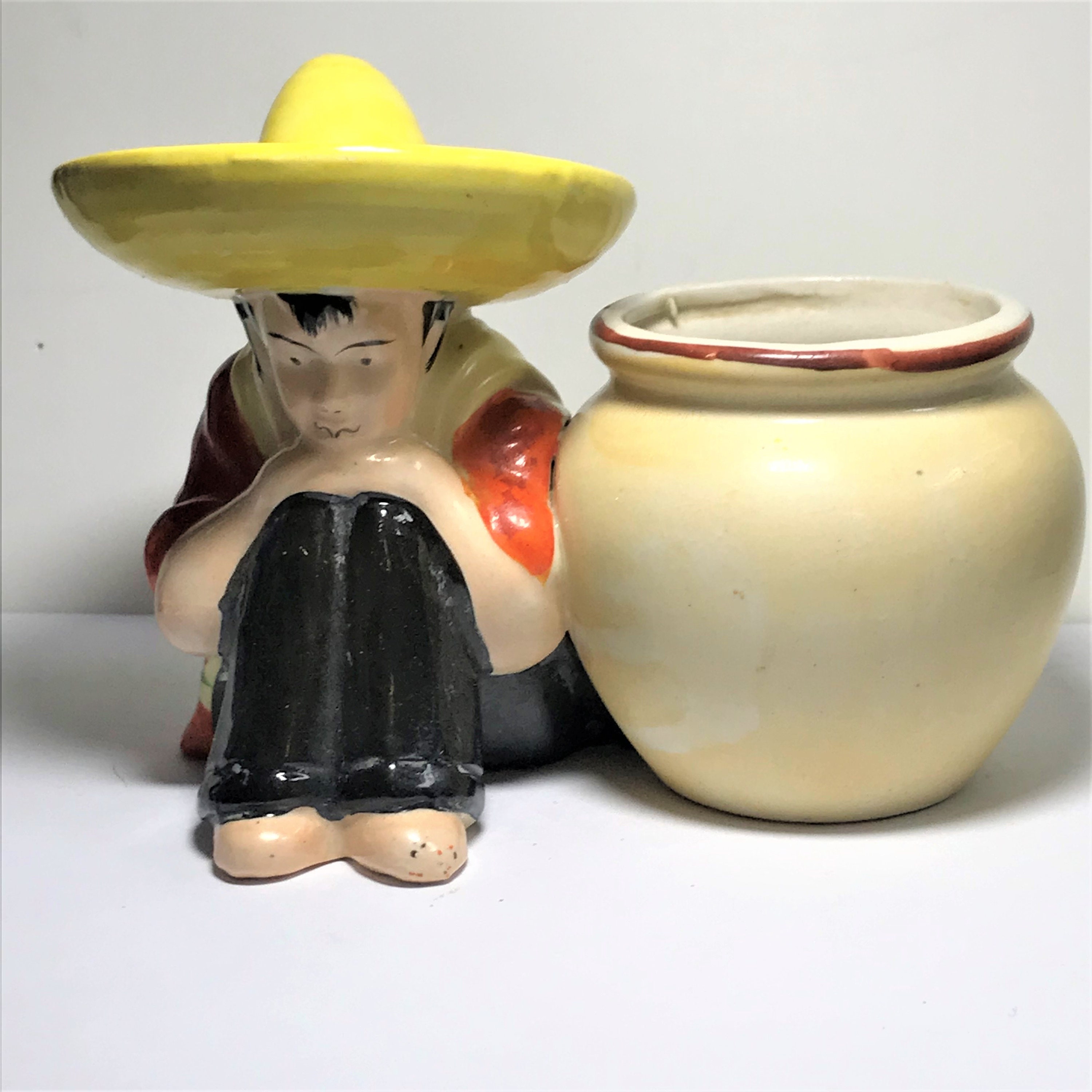A professionally photographed, antique-style ceramic sculpture depicts a young, light-skinned Mexican boy with black hair peeking out from under a wide, yellow sombrero. He wears a red and off-white shirt, black pants, and no shoes. The boy sits on a white surface, knees curled to his chest, with his hands resting on his knees and his chin on his hands, appearing deep in thought. Next to him, attached at the shoulder, is an off-white ceramic vase, nearly as tall as the boy without his sombrero. The vase is wider at the top, featuring a brown glazed rim and an indentation around its neck, making it suitable for holding flowers or a potted plant. The scene is set against a white background with good lighting, emphasizing the intricate details of this decorative knickknack, reminiscent of something you might find in a grandmother's home.